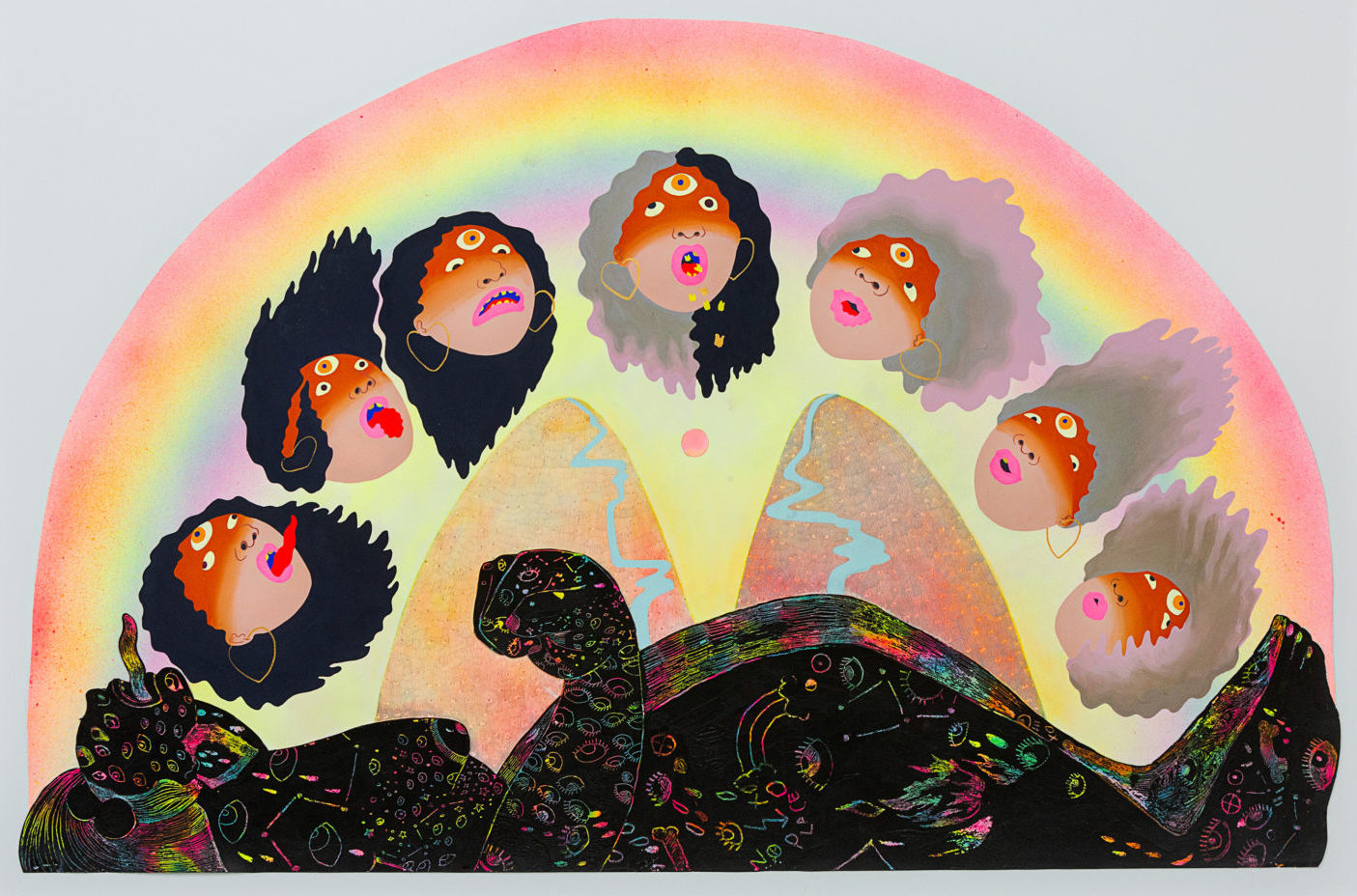The image is a fairly surreal watercolor painting set against a light gray background. It features a person lying on their back at the bottom of a rectangular frame. The person, delineated in black, has a notably rotund stomach and is adorned with colorful, swirling rainbow patterns, almost resembling rainbow writing where vibrant colors are revealed by removing a black overlay. The person's tongue, sticking out, is illustrated in a triad of blue, yellow, and red hues.

Above the person, a large, pastel-colored rainbow spans across the scene. Within this rainbow, there are seven heads with cyclopean third eyes and pink lips, each head sticking out its tongue. The heads are divided by hair color: four boast dark black hair, while three have gray hair. Some heads are adorned with heart-shaped gold earrings. An additional detail includes an orange and white emblem on the faces. The central head intriguingly has half black and half gray hair. This dreamlike and intricate composition remains unsigned and undated.